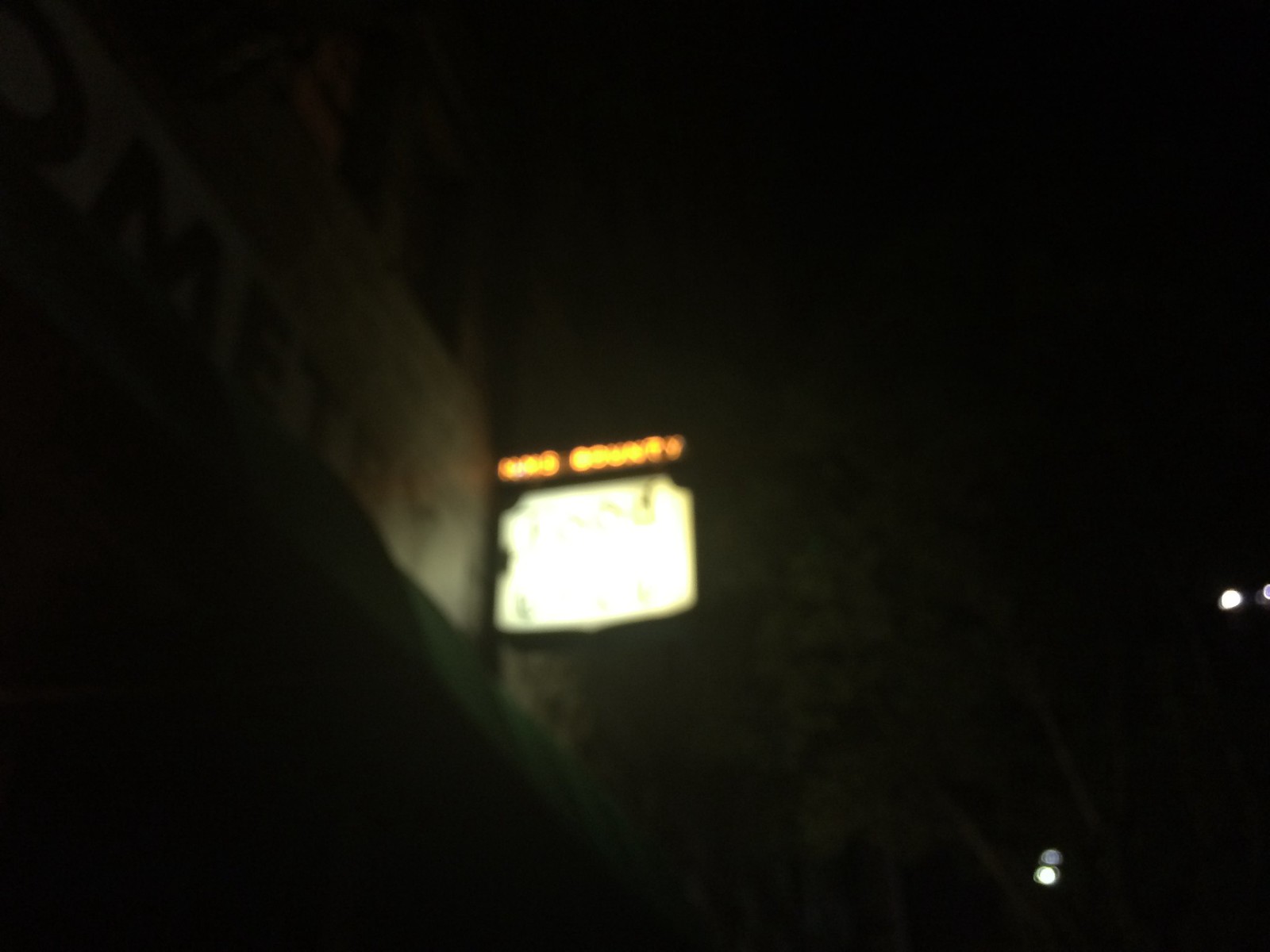This nighttime photograph, which is out of focus and slightly blurry, presents an enigmatic and shadowy scene. Dominating the left side of the image is an intensely bright, white glowing sign affixed to a building. The sign is so overexposed that its details are indiscernible, and above this blinding light, there are two words in yellow-orange text, though the blur makes them unreadable. The light emitted from the sign casts a faint illumination on the adjacent building, revealing minimal architectural features without providing clear details. Most of the photograph remains enveloped in darkness and shadow, contributing to an atmospheric and mysterious quality.